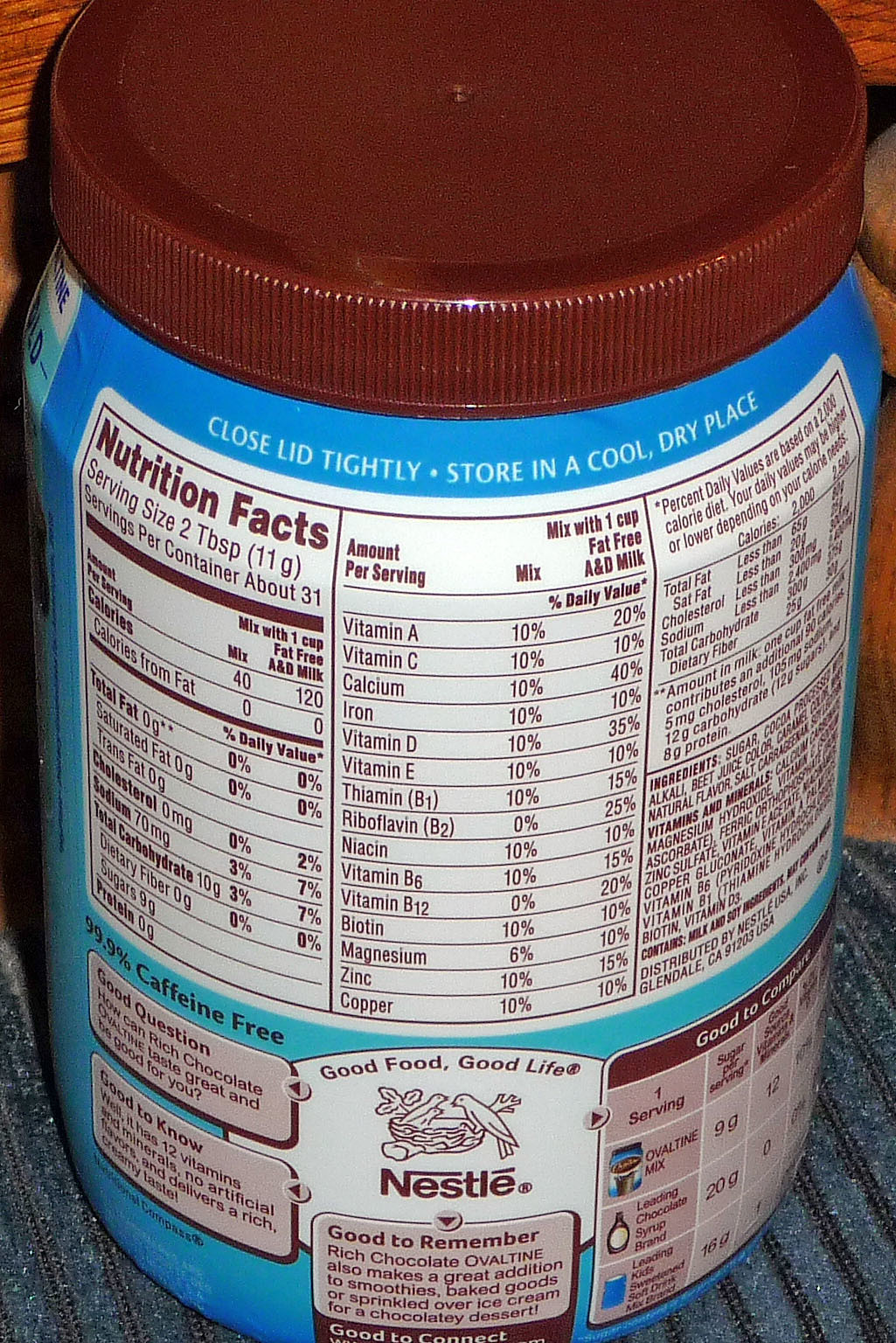The image shows the back of a round container of Ovaltine chocolate powder, topped with a brown screw-on lid. At the very top, in white text, it instructs to "close lid tightly, store in a cool, dry place." The centered brown Nestle logo is accompanied by the phrases "Good Food, Good Life," and "Good to Remember," highlighting that rich chocolate Ovaltine can enhance smoothies, baked goods, or be sprinkled over ice cream for a chocolatey treat. The nutritional label is prominently displayed, detailing the serving size of two tablespoons (11 grams), yielding about 31 servings per container. The mix is 99.9% caffeine-free, with 40 calories per serving, or 120 calories when combined with a cup of fat-free A&D milk. The label also breaks down the vitamin and mineral content, offering details both for the mix alone and when mixed with milk. The image does not show the front of the container, but the comprehensive nutritional information and guidelines are clearly visible on the back.